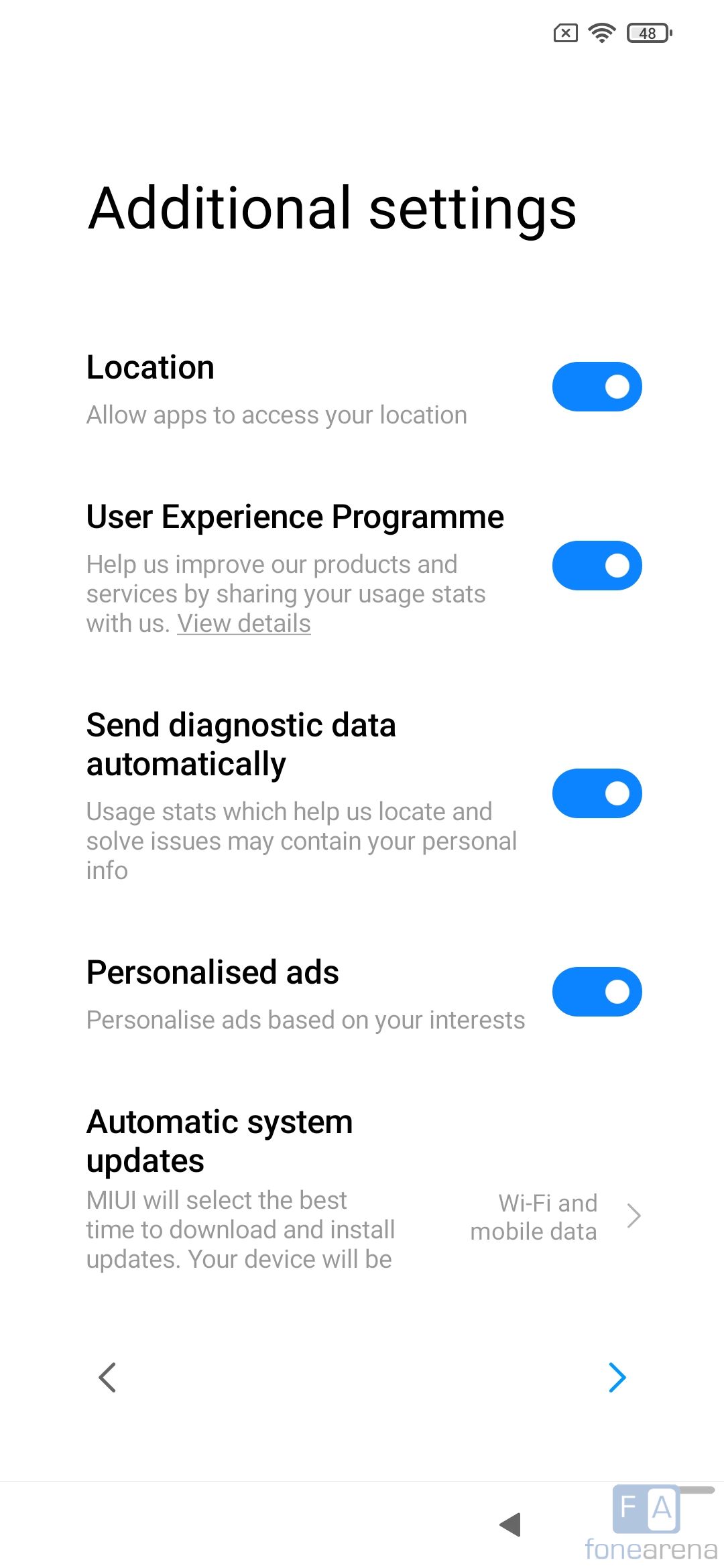This is a detailed screenshot from a mobile device's settings page. In the top-right corner, the status bar displays a rectangle with an 'X' inside, the Wi-Fi icon, and the battery icon indicating a 48% charge. The main content of the screenshot is a list of various settings and their current states:

1. **Additional Settings** section:
   - **Location**: "Allow apps to access your location" - The slider is in the on position.

2. **User Experience Program**:
   - Description: "Help us improve our products and services by sharing your usage stats with us."
   - Option: "View Details" - The slider is turned on.

3. **Send Diagnostic Data Automatically**:
   - Description: "Usage stats which help us locate and solve issues may contain your personal info."
   - The slider is in the on position.

4. **Personalized Ads**:
   - Description: "Personalize ads based on your interests."
   - The slider is turned on.

5. **Automatic System Updates**:
   - Description: "MIUI will select the best time to download and install updates. Your device will be..." (the text is cut off)
   - Mentions "Wi-Fi" and "mobile data."

At the very bottom right corner, there is an icon comprising a gray and white square divided diagonally. The left half, which is gray, contains a white 'F'; the right half, which is white, contains a gray 'A'. Below this icon, the text reads "FONEARENA."

This image captures a comprehensive view of the user’s device settings pertaining to location access, system updates, and data sharing preferences, providing a snapshot of their current configurations.